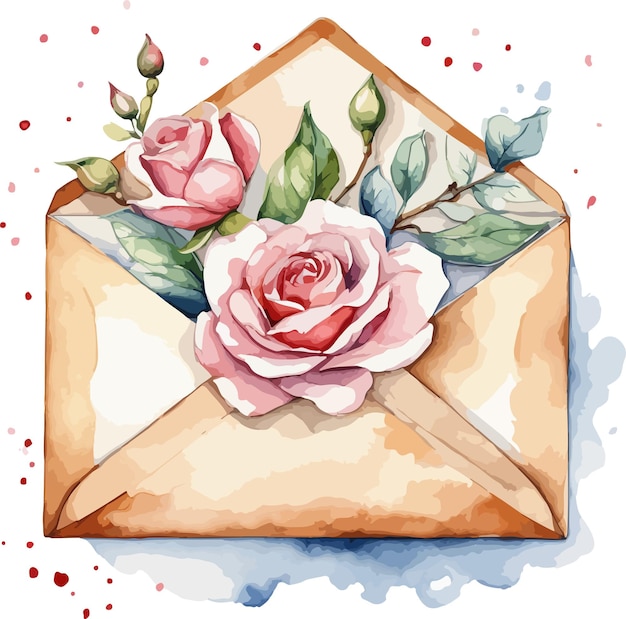The image portrays an exquisite illustration of an open, beige-colored envelope adorned with delicate watercolor details. Peeking out from the envelope are two vibrant pink roses accompanied by four rose buds, each exhibiting varied shades of green and bluish leaves. The envelope flap is lifted, revealing part of the drawn floral arrangement. Surrounding the envelope are watercolor stains in abstract blue forms, creating an artistic border. Additionally, speckles in red and pastel colors scatter around the envelope, resembling confetti, adding a whimsical touch to the composition. The overall background is white, emphasizing the elegance and romanticism of the scene.